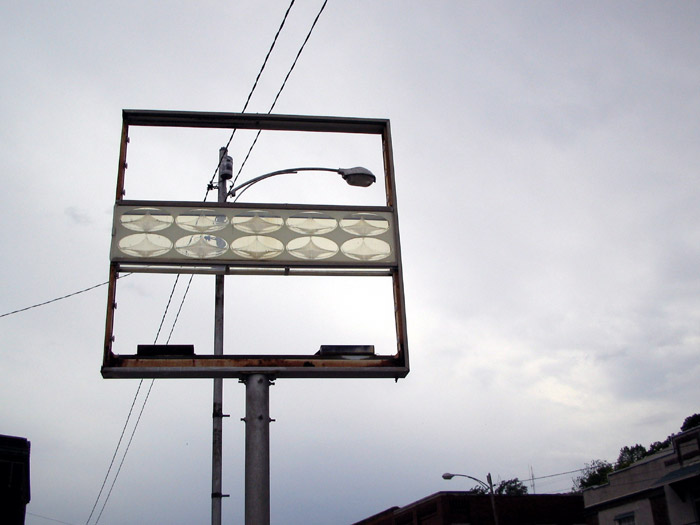This landscape-oriented photograph captures a ground-up perspective of a business street sign, characterized by its two-level structure with a decorative divider occupying roughly one-fifth of the overall height. The top and bottom sections of the sign are missing, creating transparent gaps that frame the view behind it. Through these gaps, one can observe an overcast gray sky that forms the backdrop of the image. In the immediate vicinity behind the sign, a streetlamp stands prominently, accompanied by overhead power lines that are affixed to a nearby post. The interplay of these elements creates a layered and somewhat stark urban tableau.